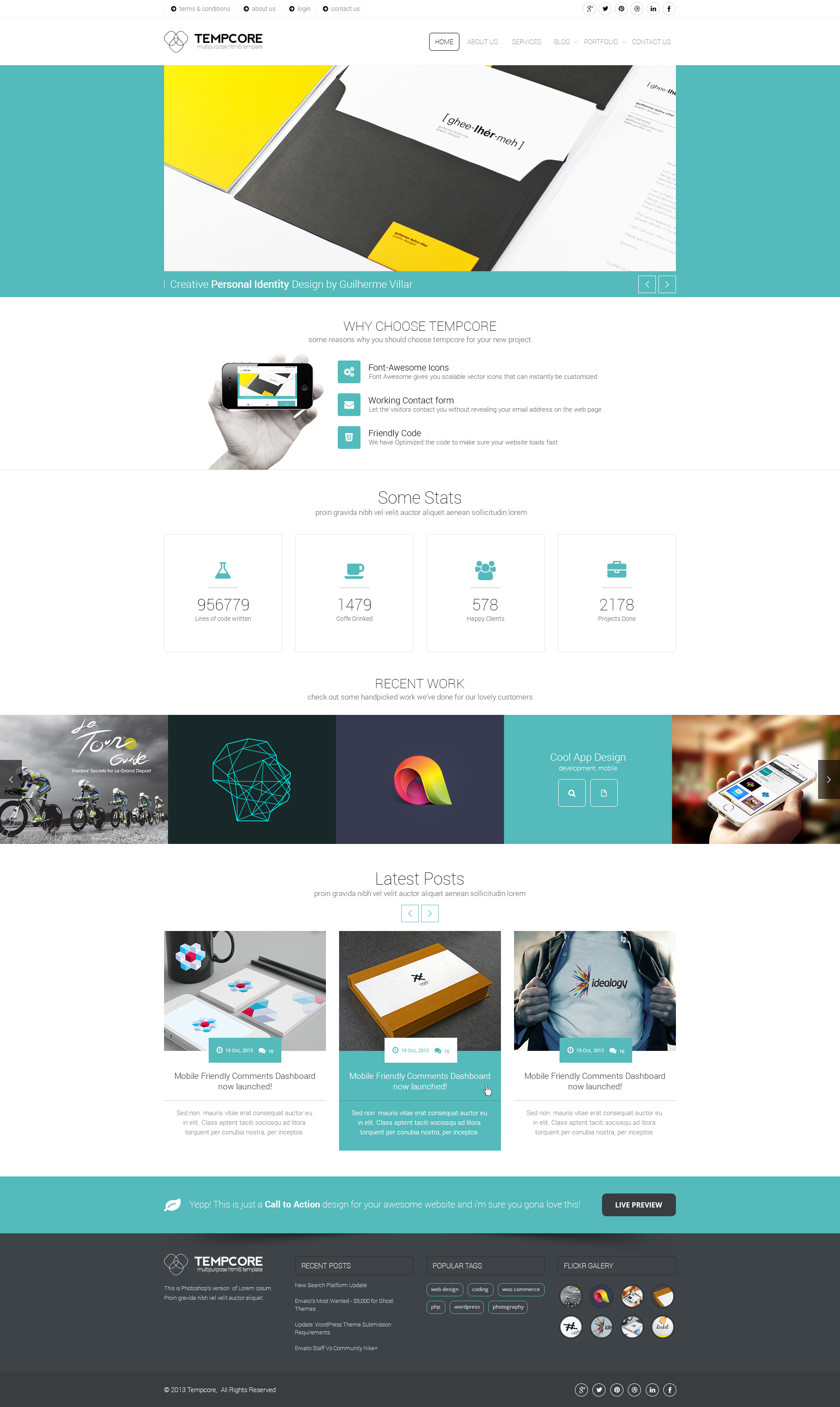The image depicts a user interface with several distinct sections. At the top, there is a teal-colored rectangle featuring a design in white, yellow, and black, accompanied by the text "TempCore." This section also includes several clickable menu items, although they are too small and blurry to discern clearly. Below this, the background transitions to white, showcasing a smartphone display that prominently features the same yellow, black, and white TempCore logo. 

Next to the smartphone image, the text "WhyChu TempCore" is displayed. Beneath this, three lines are each accompanied by a clickable teal button, although the text on these buttons is blurry and unreadable. Following this section are four white boxes, each adorned with a teal design at the top. These boxes contain text that is also too small and blurry to read clearly.

Further down the interface, there are five rectangular boxes, each containing a distinct icon. Below these, an additional three boxes, also with individual icons, are present. 

Towards the bottom of the image, a thin teal-colored rectangular bar is situated, followed by a larger black rectangular bar underneath it.